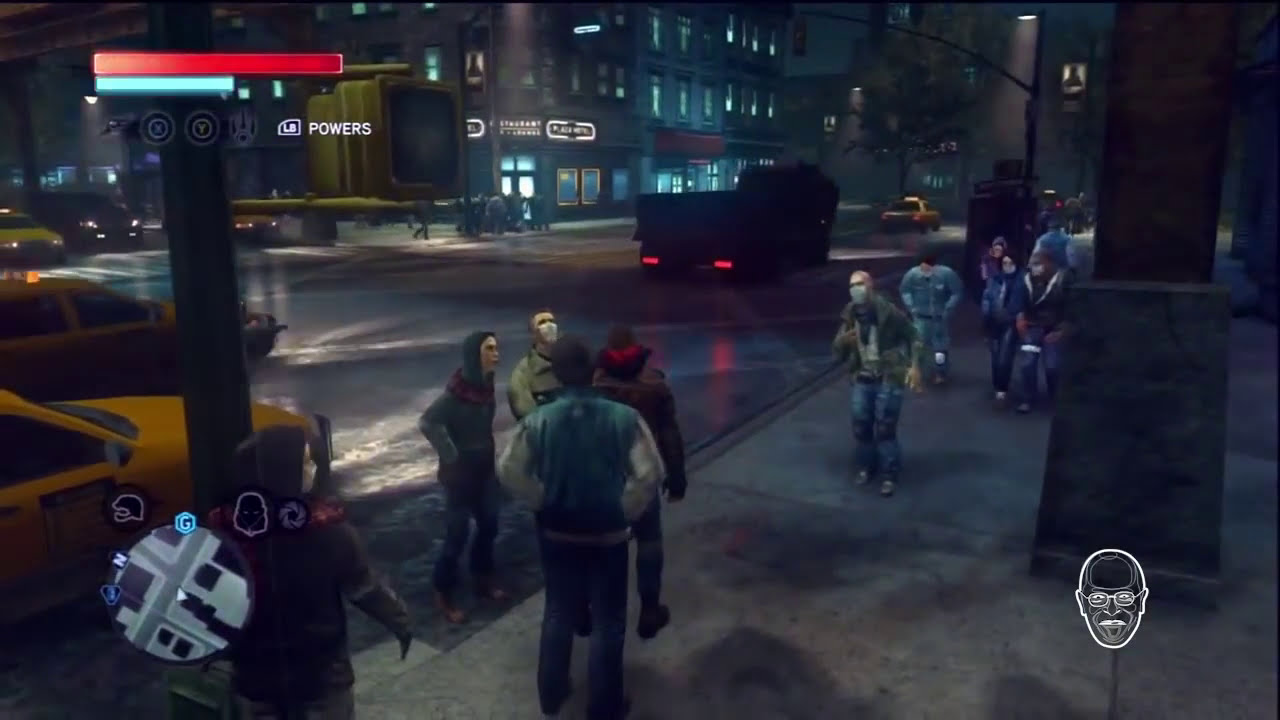This image is a detailed nighttime screenshot from a video game, depicting a bustling urban street scene. In the foreground, several characters congregate on the right-hand sidewalk, many wearing jackets and face masks, suggesting a setting influenced by a pandemic. These characters, possibly a mix of players and non-playable characters, are dressed in a variety of dark colors like browns, blues, and greens, all sporting long sleeves, indicating cooler weather.

The street, highly reflective, runs diagonally from the lower left corner to the upper right corner of the image. On this road, two yellow taxis are prominently visible, one in the lower-left corner and another further ahead. Several other vehicles, including a large truck or dump truck with bright red taillights, are seen traveling or waiting at intersections, adding to the authenticity of a busy city night. 

Illuminating the scene, glowing streetlights and the lit windows of tall buildings cast a warm glow, enhancing the urban atmosphere. Additionally, the game interface includes a mini-map in the lower-left corner, showing the player’s location within the city, and an icon of a bald man with glasses and a mustache in the lower right corner, possibly indicating the player's avatar or a character of interest. The overall color palette of the image is dark and muted, typical of a nighttime setting, brought to life by the various lights from vehicles and buildings.